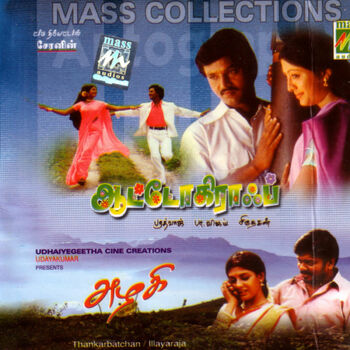The image appears to be a DVD or CD cover for a collection of possibly Hindi movies or music, given the presence of various traditional outfits and the phrase "mass collections" prominently displayed at the top. The background features a gradient of blue with mountains and fog leading down to meadowy hills, creating a serene backdrop.

In the top section of the image, a man with dark skin wearing a white bandana shirt and a woman in a pink dress, both holding a pole, are looking down. The same pair appears on the left-hand side, now dancing; the man has his white bandana shirt open to reveal a red shirt underneath, and the woman has changed into a red-pink dress.

In the bottom right corner, another couple is illustrated. The woman, in a traditional orange dress, seems to be crying while a man in a purple-pink bandana shirt comforts her, his hand on her cheek and her hand holding his.

There are also additional details like an author's name to the upper left of the "mass collections" banner and some additional text in various vibrant fonts, possibly in an Indian language, adding to the cultural context of the collection.